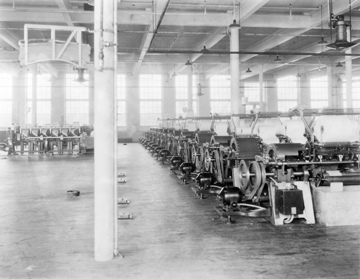This detailed black and white photograph captures the interior of an old factory, showcasing rows upon rows of identical machinery, possibly textile or printing equipment. The machinery, organized in parallel lines, stretches from the foreground on the right all the way to the back of the room and also spans horizontally in the distant background. Large white rolls, likely paper or fabric, rest atop the machines, accentuating the industrial atmosphere. The floor, appearing to be spotless concrete, features prominent metal pillars supporting the ceiling. The ceiling itself is outfitted with hanging lights and visible pipes, contributing to the historical industrial aesthetic. On the far side of the room, numerous large windows extend from the top to the bottom, flooding the area with natural sunlight and reinforcing the historical feel of the space. Despite the aged quality of the photograph, which confirms its authenticity, the factory space appears exceptionally clean and well-maintained.